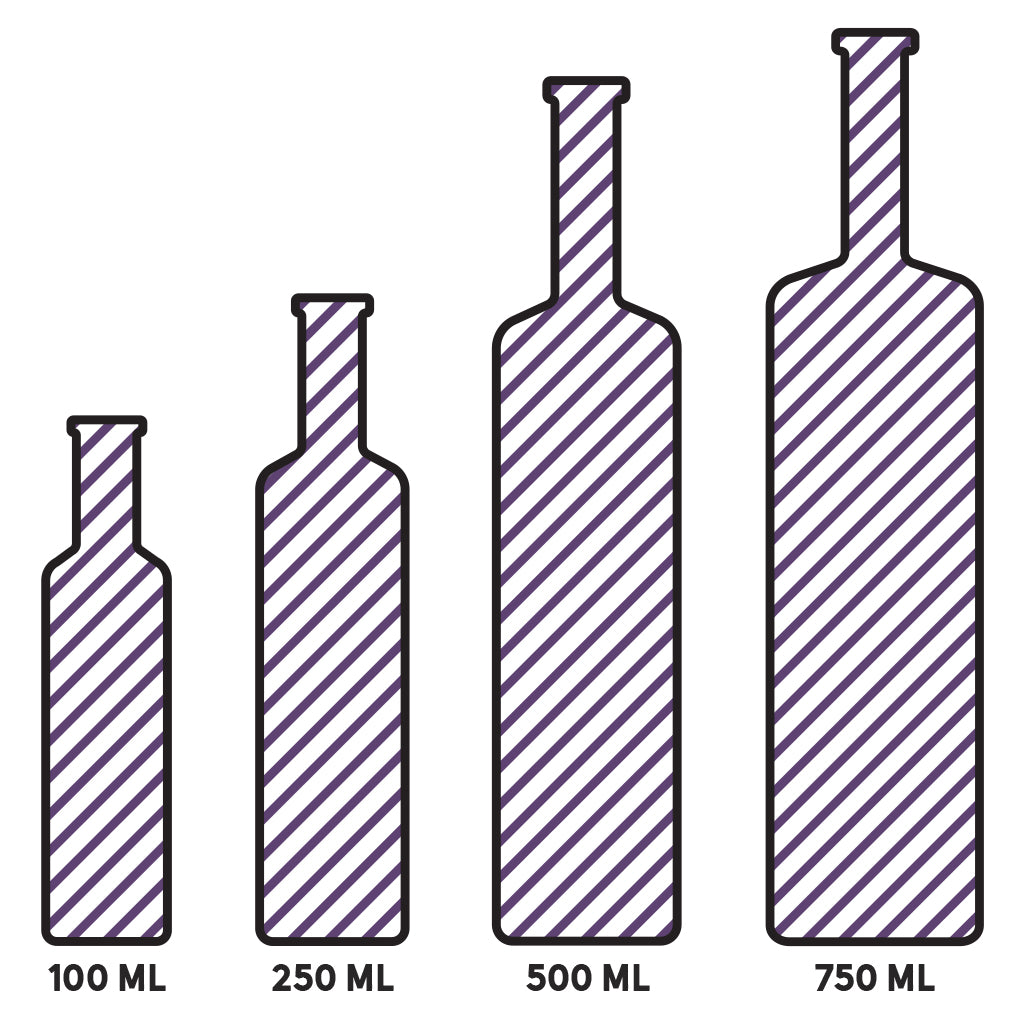This black and white image depicts the outlined sketches of four bottles, each progressively larger and labeled with their respective sizes: 100 milliliters, 250 milliliters, 500 milliliters, and 750 milliliters. The outlines of the bottles are drawn with a black border, and each bottle features diagonal lines, going from the lower right to the upper left. These lines, possibly intended to be blue as noted in one description, traverse upwards from the base to the mouth of the bottles, giving a sense of uniform texture. The bottles, resembling wine or possibly liquor bottles, are arranged from smallest to largest, left to right, on a plain white background. Each bottle also features a small lip at the top, adding to the accuracy of their depiction.